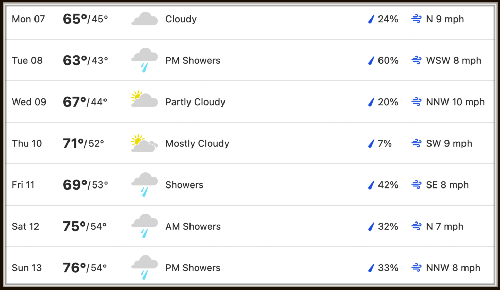This image represents a weather forecast platform displaying detailed weather information for an entire week. 

On the top left, organized vertically, the current week’s dates are listed starting with Monday, the 7th. Adjacent to each date, the forecast for the respective days is presented. 

- For Monday, 07, the high temperature is marked as 65°F and the low at 45°F, illustrated in bold black text. Directly beside these numbers, a cloud icon with the word "Cloudy" indicates overcast conditions. Further to the right, two additional pieces of information are displayed: humidity at 24% and wind speed and direction as N at 9 mph.

- Moving to the second row for Tuesday, 08, the forecast specifies 63°F as the high and 43°F as the low. A cloud icon with raindrops signifies "PM showers." The chance of precipitation is noted at 60%, with winds coming from the WSW at 8 mph.

The pattern continues similarly for the remaining days of the week, from Wednesday, 09, to Sunday, 13. The respective weather conditions vary, including descriptors such as "Partly Cloudy," "Mostly Cloudy," "Showers," "AM Showers," and "PM Showers."

Towards the bottom right corner, further details are provided, including another wind direction and speed noted as North-Northwest at 8 mph. This detailed layout allows viewers to easily comprehend the week’s weather outlook at a glance.